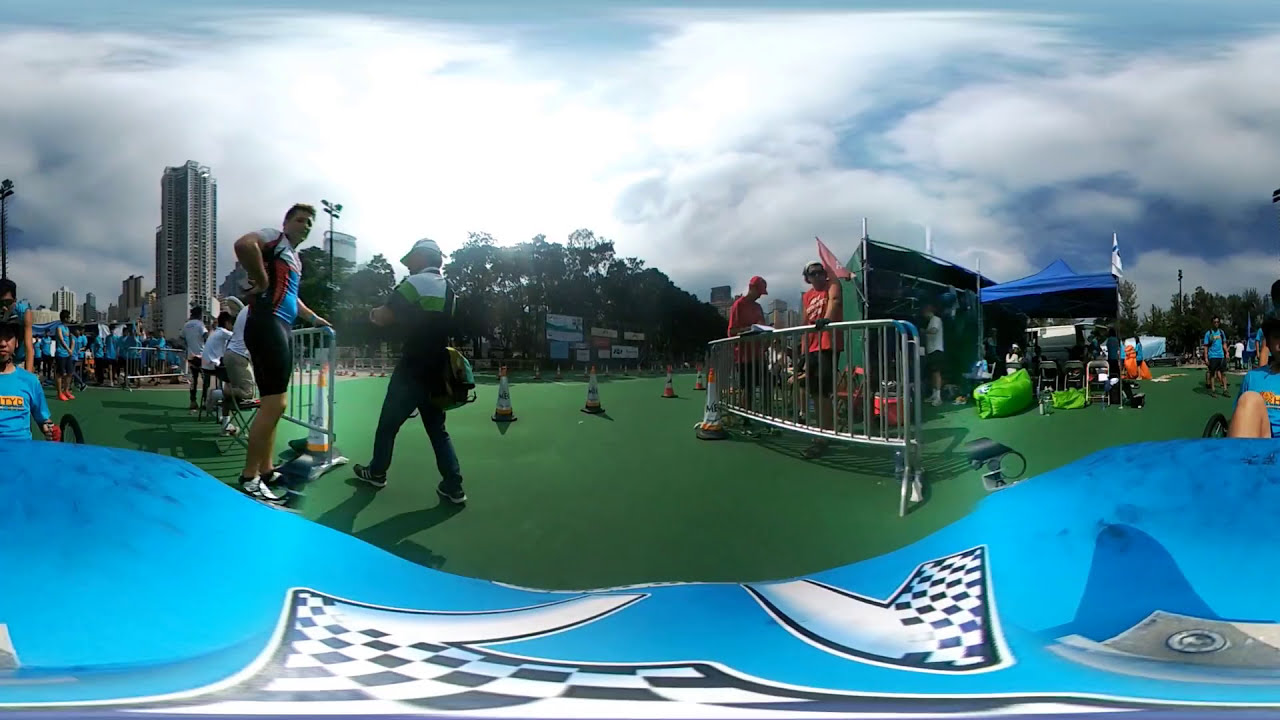The image captures a lively 360-degree outdoor sporting event, possibly a race or a competition involving pedal-powered vehicles. Dominating the scene is a young boy in a low, blue pedal car adorned with various designs and checkered flags at the front, positioned on a green AstroTurf track. The track is marked with orange cones, guiding participants along their path. Spectators and participants alike scatter the area, with some people elevated above the boy, hinting at seating or standing positions higher than the vehicles. A cattle fence runs along both sides of the track. On the right, two men in red t-shirts stand behind the fence, while on the left, a man in a blue, red, and black biking outfit stands with his hand on his hip, next to another individual in black pants, a green and white shirt, and a white hat. The venue is bustling with activity, featuring several tents and gazebos—one green and another blue—occupied by workers. The background showcases a line of trees and the outline of a cityscape with a notable tall skyscraper to the left. Above, the sky is a patchwork of blue and white clouds, encapsulating the vibrant atmosphere of the event.